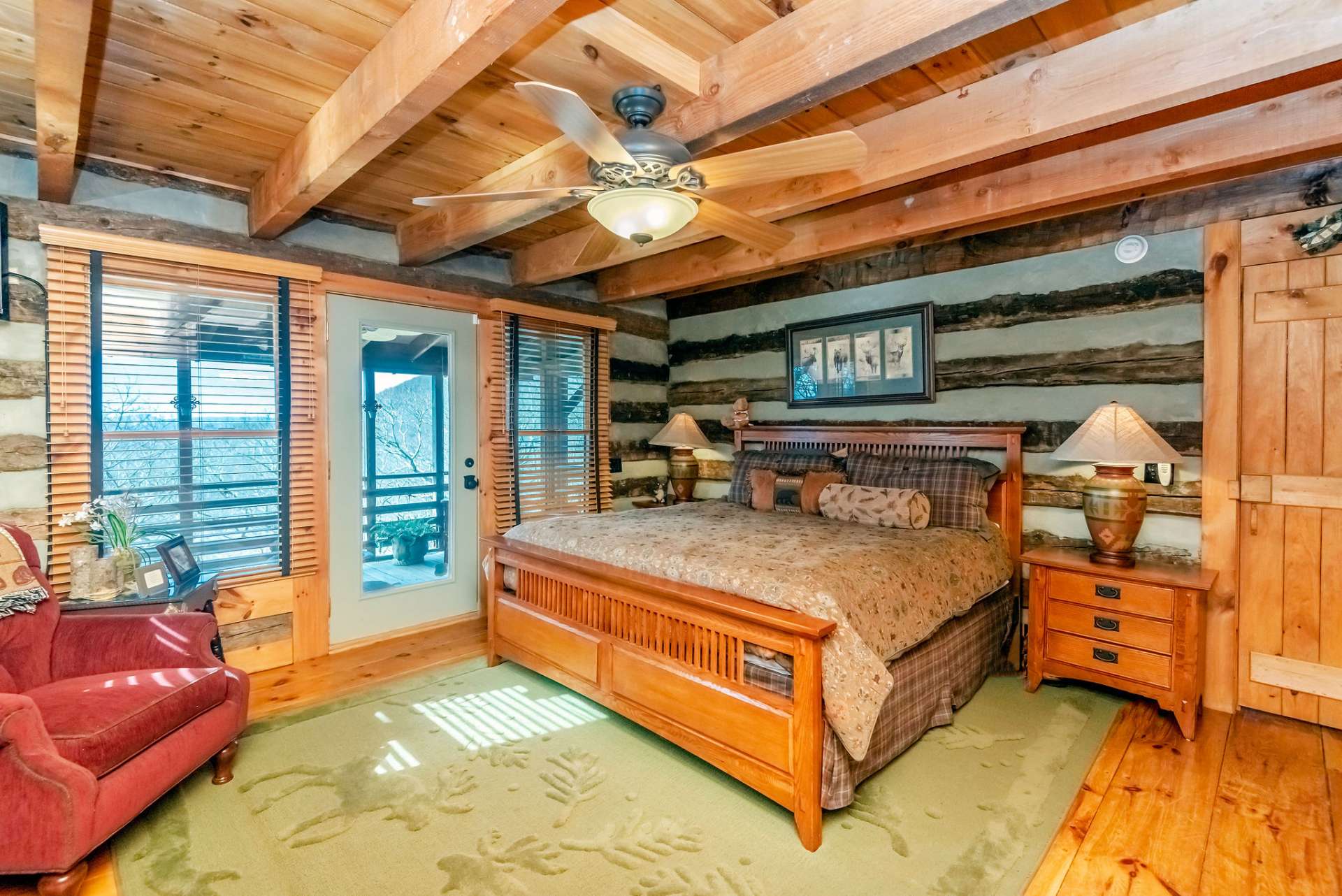This image is of a beautifully detailed bedroom, likely in a log cabin home or resort. Dominating the center of the room is a king-size bed with a rustic wooden frame, adorned with a white comforter featuring a brownish floral pattern. The bed is complemented by tan and brown plaid pillows and shams. The hardwood floor is partly covered by a light green area rug adorned with moose designs. 

On either side of the bed are wooden nightstands with brass-colored lamps featuring off-white shades. One nightstand includes a switch bar with an AC remote, and the wall behind the bed holds a painting in a rectangular black frame. The wooden ceiling boasts wooden beams and a designer ceiling fan with four blades and attached lighting. 

To the left of the bed, there is a glass-paneled door leading to a balcony with railings and indoor plants, offering a scenic view of a hilly, wooded area. The room is brightened by sunlight streaming in through the open shades of the windows flanking the door. 

On the bottom left, a plush red cushiony chair or recliner adds a splash of color and comfort. A side table near the chair holds photo frames and a flower vase. The warmth and natural charm of the wooden design, from the ceiling to the floor, make this room a quintessential cozy cabin retreat.